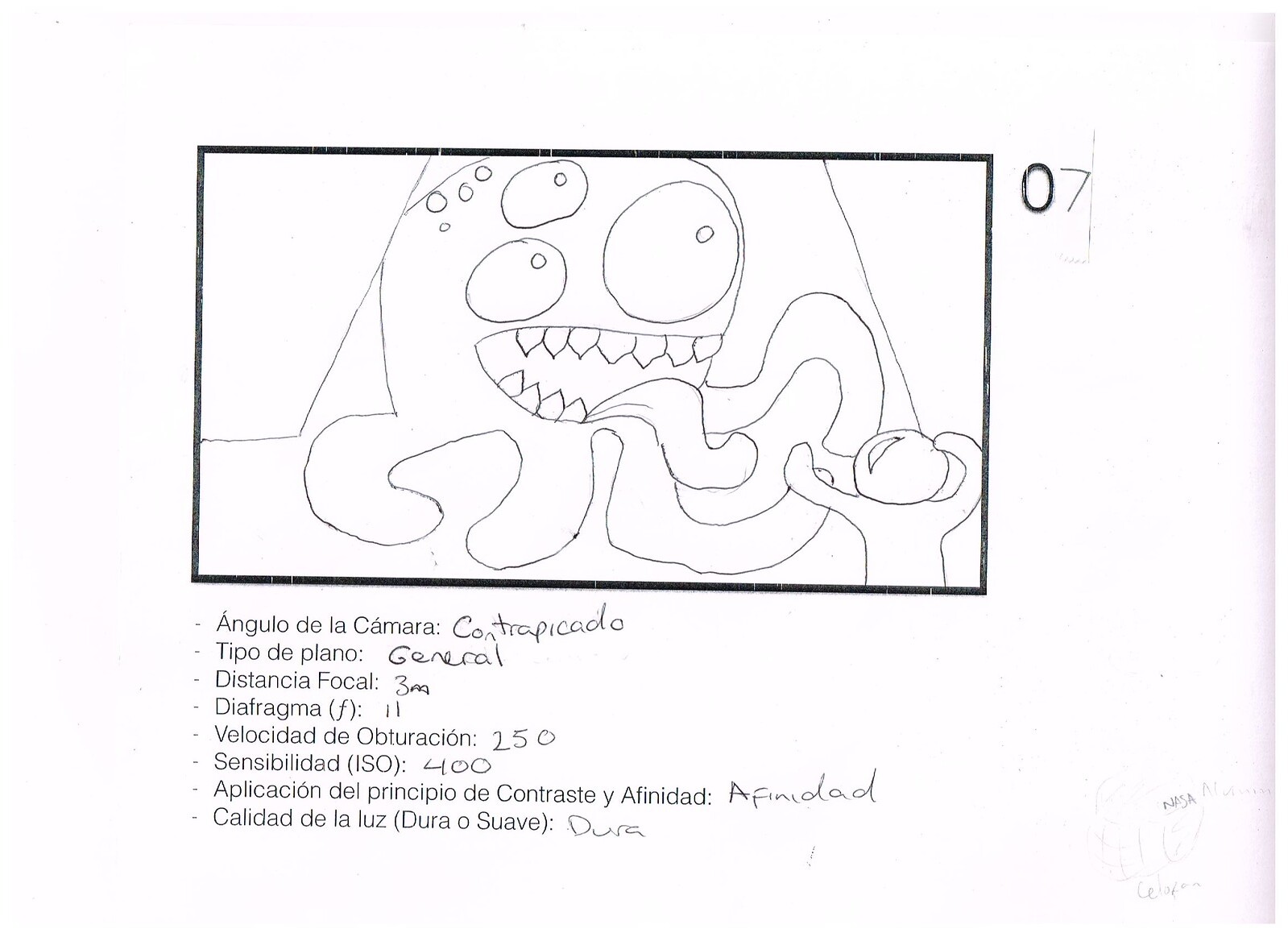The image features a black-ink sketch within a rectangular frame on a white page, labeled "07" at the top right corner. The drawing depicts a fantastical octopus-like creature with four legs, a gaping mouth filled with numerous teeth, and two tongues sticking out. It has three eyes—one large eye on the right and two smaller ones, one above the other, on the left—with three dots on its head. The creature appears to be menacing a person in the bottom right corner, who is raising their arms in fright. Below the sketch, there is text mostly in Spanish, divided into printed and handwritten sections, detailing various camera settings and descriptions. Key points include "Angelo de la Camara," "Contra Picado," "Tipo de Plano: General," "Distancia Focal: 3M," "Diafragma (F): 11," "Velocidad de Obturación: 250," "Sensibilidad (ISO): 400," "Aplicación del Principio de Contraste y Afinidad," and "Calidad de la Luz (Dura)." The printed text is on the left and handwritten annotations in ballpoint pen are on the right.